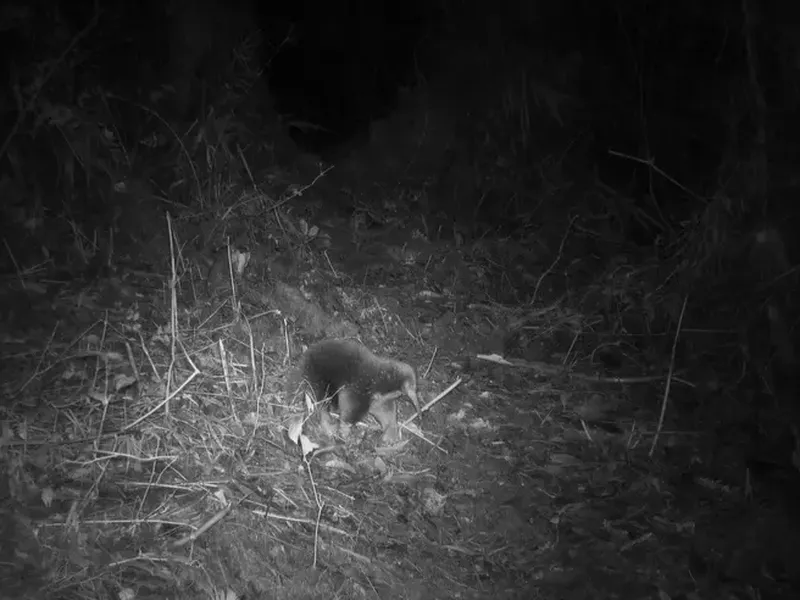This striking black-and-white night vision photograph, likely captured by an outdoor surveillance camera, vividly depicts an anteater traversing a forest. The anteater, its elongated snout prominently visible, is bathed in the radiant glow of a motion-activated light, starkly illuminating its fluffy fur and four sturdy legs against the pitch-black backdrop. In the foreground, illuminated by the same light, lie scattered broken branches, leaves, and a dirt-laden ground, adding texture and context to the scene. The scene suggests an anteater in motion, potentially seeking out its next meal, using its characteristic long tongue to extract ants and insects from holes in the earth.